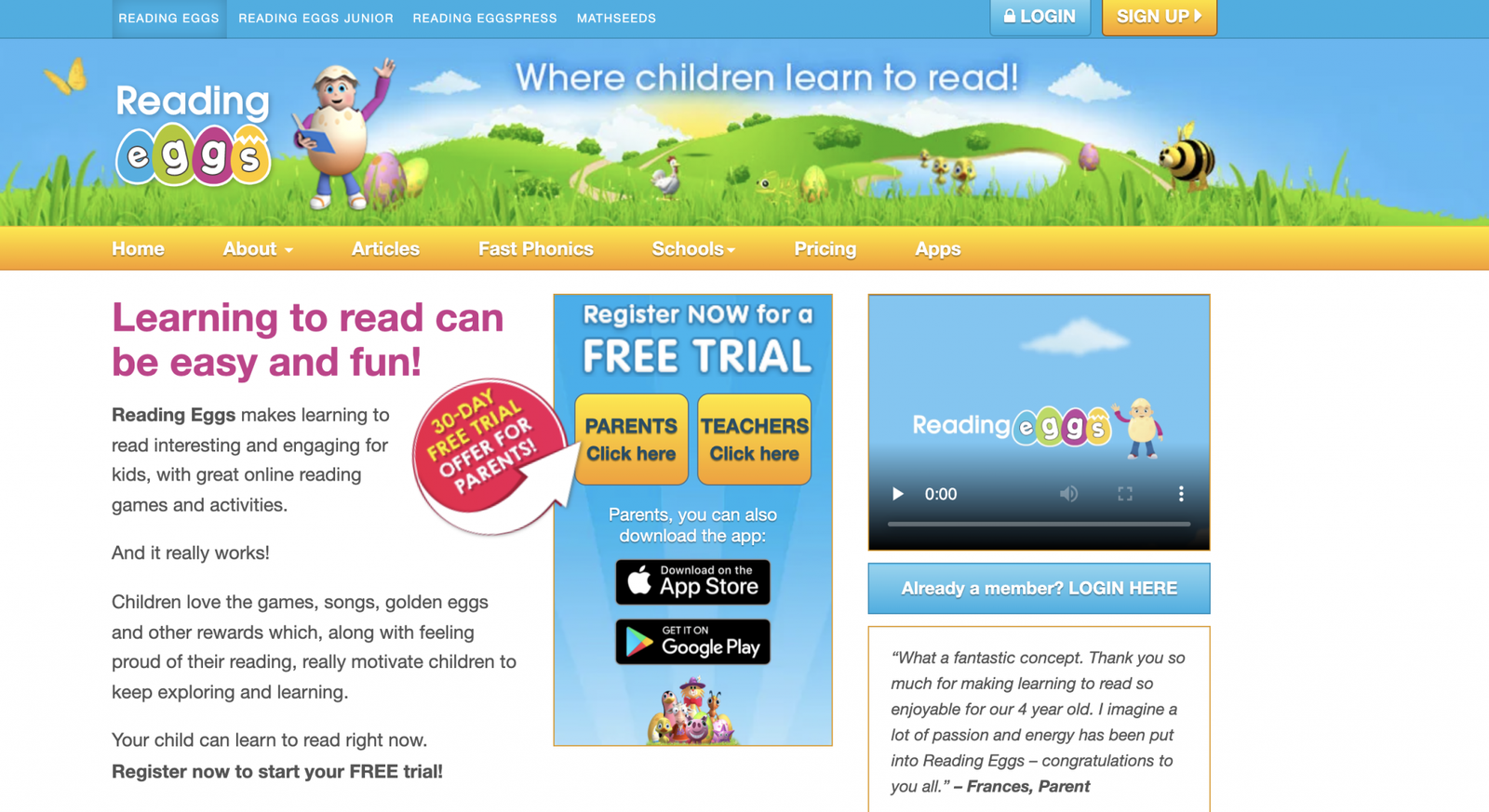The image displays a white tab at the top containing the words "Reading Eggs" and "Reading Eggs Junior," highlighted to emphasize these terms. Below, there are two rectangular buttons: the first one is blue with "Log In" written in white, and the second button features a gradient of orange to yellow, also stating "Log In" in white. An orange butterfly icon is positioned next to the text "Reading Eggs," followed by the phrase "Children learn to read."

Underneath these elements, there's an orange-bordered section with various navigation options in white text: "Home," "About," "Articles," "Products," "Schools," "Prices," and "Ads." The background transitions to a purplish-magenta color with the heading "Learning to read can be fun and easy" in white. 

The main body text is in black and reads, "Reading Eggs makes learning to read interesting and engaging for kids with great online reading games and activities, and it really works. Children love the games, rewards, and always feel proud of their reading achievements, which motivate them to explore and learn more. Your child can start learning to read right now. Register now to start your free trial."

Towards the bottom, a red circle contains a yellow banner stating "30-day free trial offer for parents" in white. It encourages users to "Register for a free trial" and mentions the app's availability for download on the App Store and Google Play.